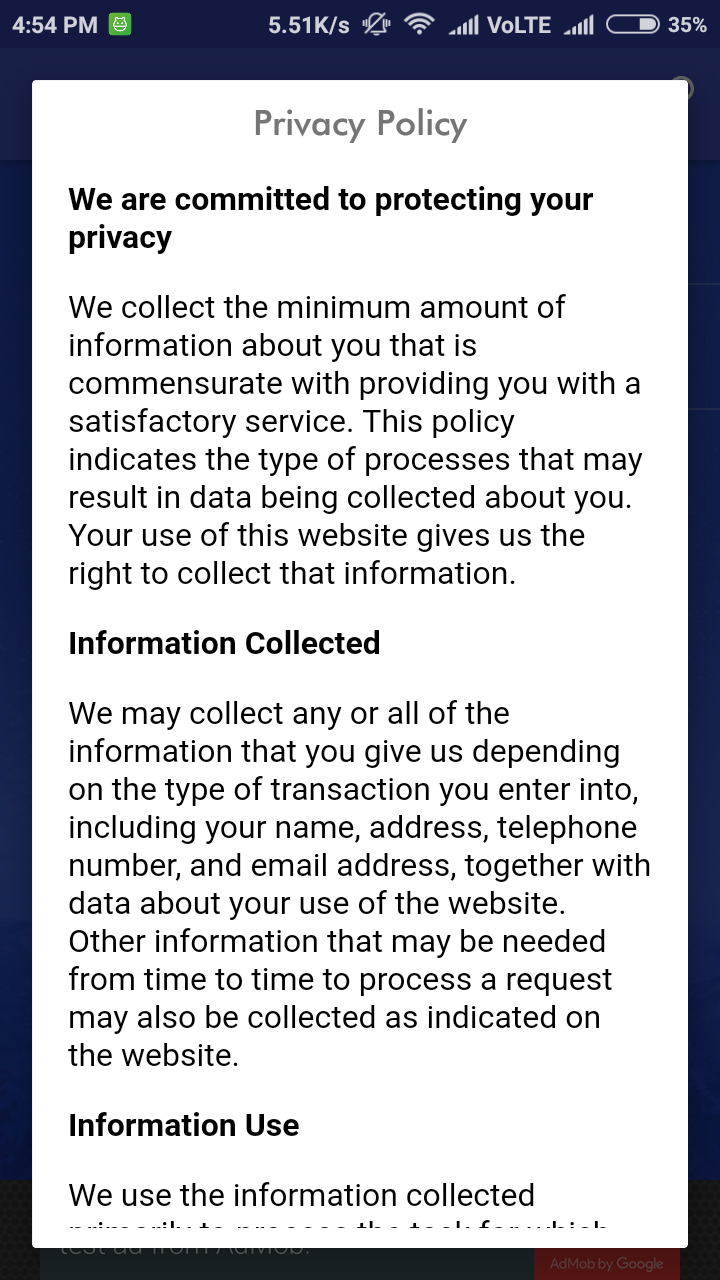The image showcases a privacy policy pop-up on an Android smartphone, displaying around 35% battery life and full signal bars. The privacy policy, shown in a neatly organized format, emphasizes the service's commitment to protecting user privacy. It outlines that only the minimum necessary information is collected to provide satisfactory service. The document details the types of data gathered, such as the user's name, address, telephone number, and email address, along with usage data from their interactions on the website. This collected information is used to process requests and improve service quality. Although the pop-up implies the collection of comprehensive user data, it also hints at the potential use of this data for profit purposes. The tone of the document suggests a thorough but somewhat invasive data collection strategy, underlying the complex trade-off between service convenience and personal privacy.